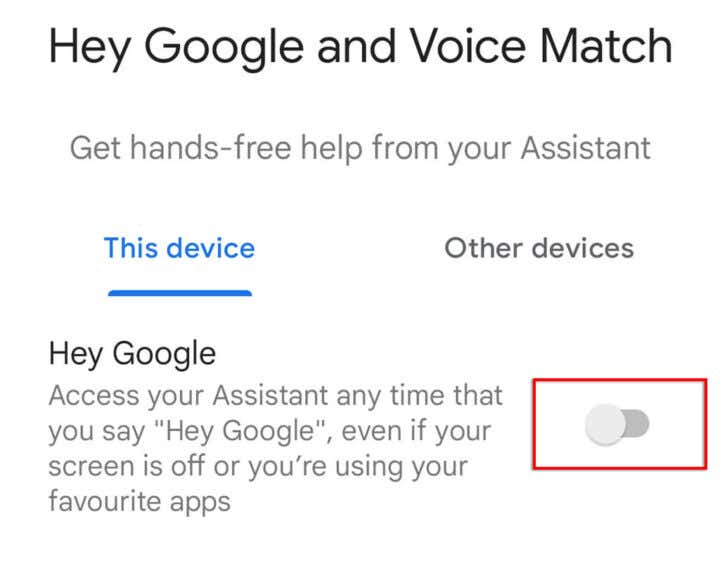The image features a clean, white background with a centered interface detailing Google Assistant settings. At the top, black text displays "Hey Google" and "Voice Match" prominently. Directly below, gray text reads, "Get hands-free help from your Assistant."

Two categories are shown beneath this text: "This Device" on the left, which is highlighted in blue and underlined, and "Other Devices" on the right. Further down, in black text, it says, "Hey Google," followed by gray text explaining, "Access your Assistant anytime you say 'Hey Google,' even if your screen is off or you're using your favorite apps."

To the right, a toggle switch is positioned within a red rectangle, currently indicating that the feature is off by appearing gray.